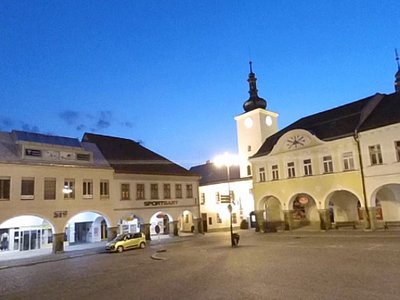This image captures a tranquil town square at twilight, featuring a series of white buildings with prominent archways along the lower levels, likely housing shops. The upper levels are characterized by numerous windows, suggesting residential use. On the left side of the square stands a white building with an illuminated storefront, marked by multiple well-lit archways, and a greenish small SUV parked in front of it. A notable feature at the far end of the square is a large white steeple with a black pedestal, topped with a cross that reaches into the darkening sky. This steeple, possibly part of a church, is accompanied by a round window beneath it. A streetlight at the corner of the square brightly illuminates the area, ensuring the surrounding buildings are well-lit. In the backdrop, additional buildings with similar architectural features extend the quiet charm of the setting.